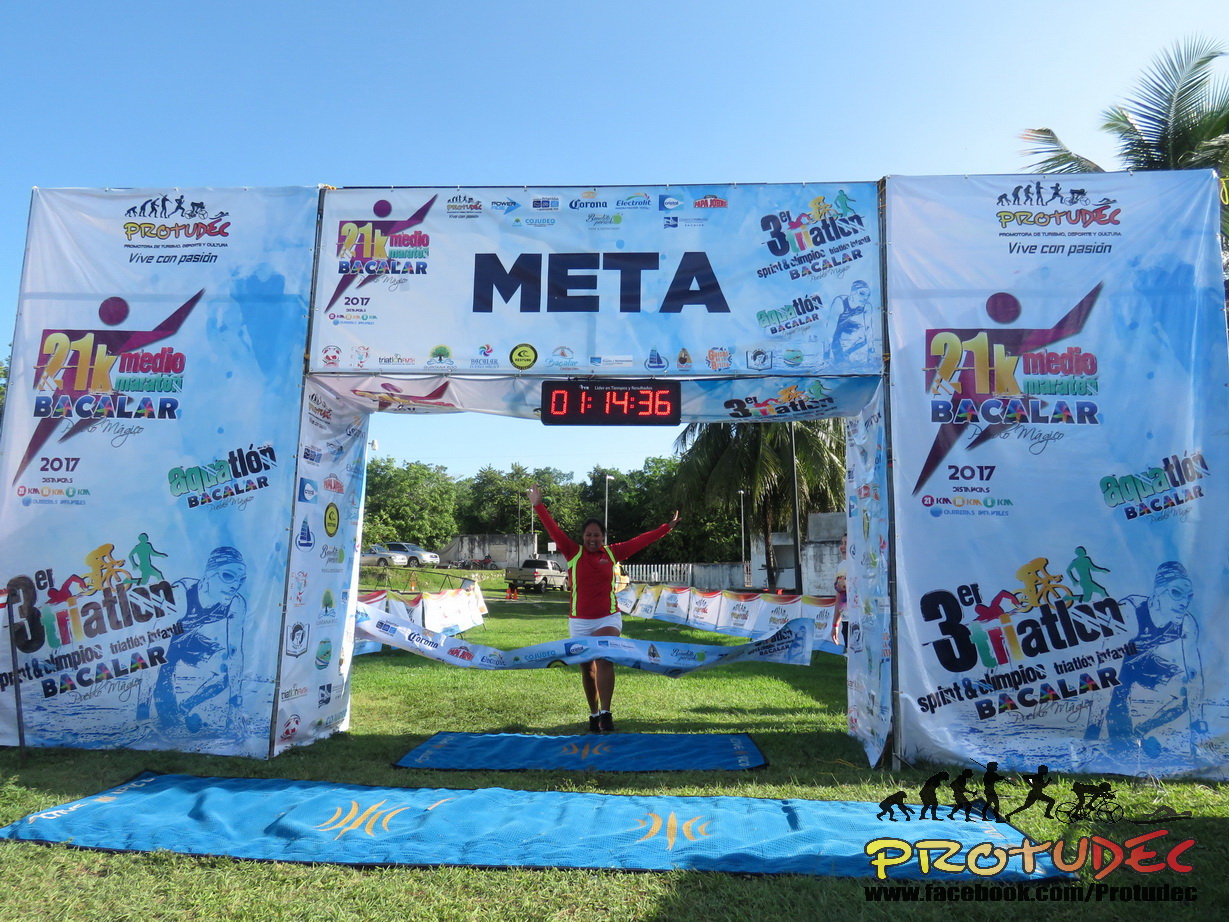In the photograph, a woman, possibly finishing first, is seen triumphantly crossing the finish line of an outdoor race. The event takes place under clear blue skies amidst lush green grass and vibrant foliage, with numerous palm trees in the background. A large pavilion with metal tubing and white canvas displays various advertisements and sponsors, highlighted with a prominent "META" sign and the text "Baccalaureate 21K Media Marathon." The pavilion also features a digital clock prominently showing a time of 1 hour, 14 minutes, and 36 seconds. The runner, dressed in a long-sleeve red shirt accented with neon yellow stripes and white shorts, raises her hands in celebration as she breaks through the banner draped at knee height. Blue tarps or towels can be seen on the ground ahead of her. In the lower right corner, additional text reading "Proto Pro to Deck" and an evolution-themed image illustrate the progression from monkey to primate, hunter, runner, and cyclist.